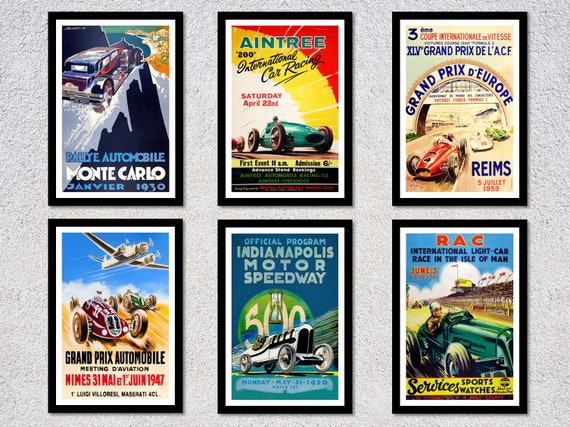The image showcases a series of six vertically aligned, framed posters mounted on a wide, vertical gray wall. Each poster is rectangular with black frames and white trim. Starting at the top left, the first poster reads "Automobile, Monte Carlo, Janvier 1930" and features a 1930s hot rod descending a slope. To its right is a poster that announces, "Aintree, International Car Racing, Saturday, April 22nd", promoting a vintage car race. 

Next in line is the "XLV Grand Prix de l'ACE, Grand Prix de Europe, REIMS, 5th of July 1959", highlighting a significant European race. Below that, on the bottom left, is the "Grand Prix Automobile, Meeting de Aviation, Nîmes, 31st of May to 1st June 1947", showing a plane flying over the car race. Moving right, the fifth poster advertises an "Official Program, Indianapolis Motor Speedway 500", marking an iconic American motor racing event.

Finally, the bottom right poster is for the "RAC International Light Car Race in the Isle of Man", rounding out this collection of classic automotive racing advertisements.